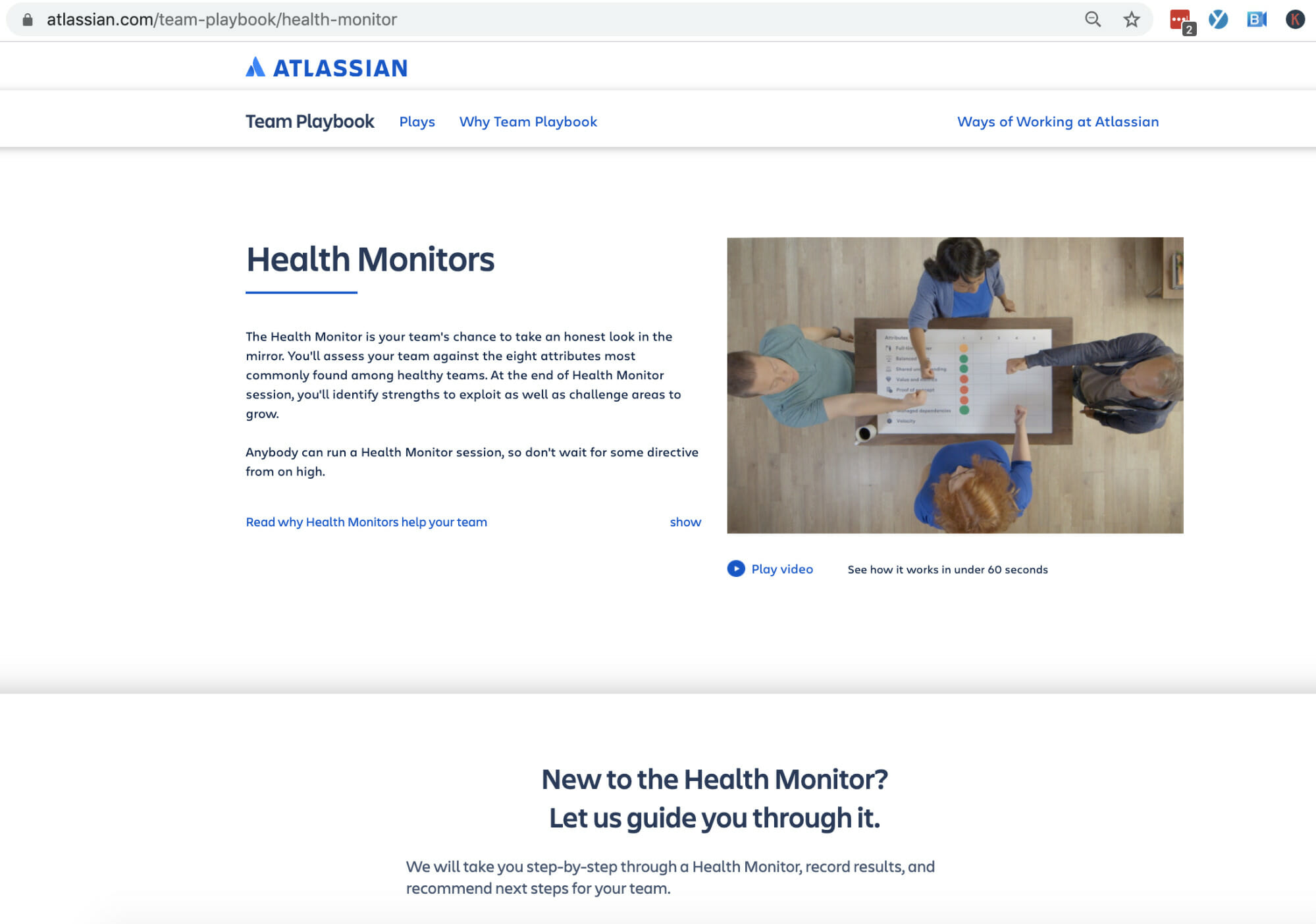This photo captures a computer screen displaying the Atlassian website, specifically the "Team Playbook | Health Monitor" page. The website features a clean, white background with the Atlassian logo prominently displayed in blue lettering at the top left corner. Directly below the logo, navigation links read "Team Playbook," "Plays," "Why Team Playbook," and on the right side, "Ways of Working at Atlassian."

The main content area showcases an article on "Health Monitors," which emphasizes their importance for teams to self-assess and improve. The article notes: "The health monitor is your team's chance to take an honest look in the mirror. You'll assess your team against the eight attributes most commonly found among healthy teams. At the end of the health monitor session, you'll identify strengths to expand as well as challenge areas to grow. Anybody can run a health monitor session, so don't wait for some directive from on high. Read why health monitors help your team."

Accompanying the text is an image on the right side, depicting four people engaged in a teamwork session around a table. Below the image, a button invites users to "Play Video" to see how the health monitor works in under 60 seconds. At the bottom of the page, there's a prompt for those new to Health Monitor: "Let us guide you through it. We will take you step by step through a health monitor, record results, and recommend next steps for your team."